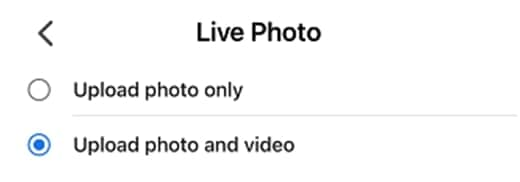The screenshot features a minimalist user interface on a white background. In the top left corner, there's a small chevron icon pointing to the left, indicating a back button. Adjacent to the chevron is some white space followed by the text "Live Photo" in black.

The main section of the screenshot displays two selectable options, each accompanied by a circular radio button. The first option, which is not selected, features an empty white circle and is labeled "Upload Photo Only." Below this, there is a light gray horizontal line that separates the first option from the second.

The second selection consists of a blue circle containing a blue dot in its center, indicating that it is the active choice. This option is labeled "Upload Photo and Video." The rest of the screen is blank, filled with white space, preserving the simple and uncluttered design.